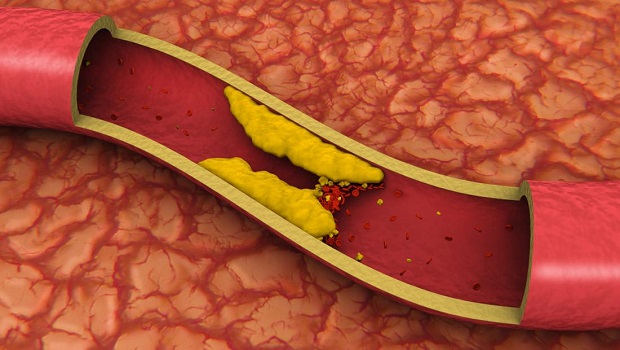The image is a detailed 3D rendering of a clogged artery, showcasing the process of arterial blockage likely caused by cholesterol or fat in the bloodstream. Central to the image is a long, red tube, representing the artery, with a cross-sectional cutaway revealing its interior. Inside the artery, the red liquid signifies blood flow, while the inner walls appear yellow, highlighting the accumulations of plaque. Prominent in the rendering are two large masses of yellow gunk, referred to as plaque, obstructing either side of the artery. This obstruction creates a traffic jam for the numerous round red blood cells attempting to pass through, resulting in a significantly narrowed passage. The artery wall, visible through the cutaway section, is distinctly yellow in contrast to the red interior. The background features a textured, skin-like surface with small wrinkles and tiny veins, adding to the realism of the biomedical illustration. The overall depiction emphasizes the severe blockage and the resultant congestion within the artery, providing a vivid representation of what can lead to heart attacks. Various smaller yellow and red dots can also be seen on one side of the artery, further illustrating the clogged condition.